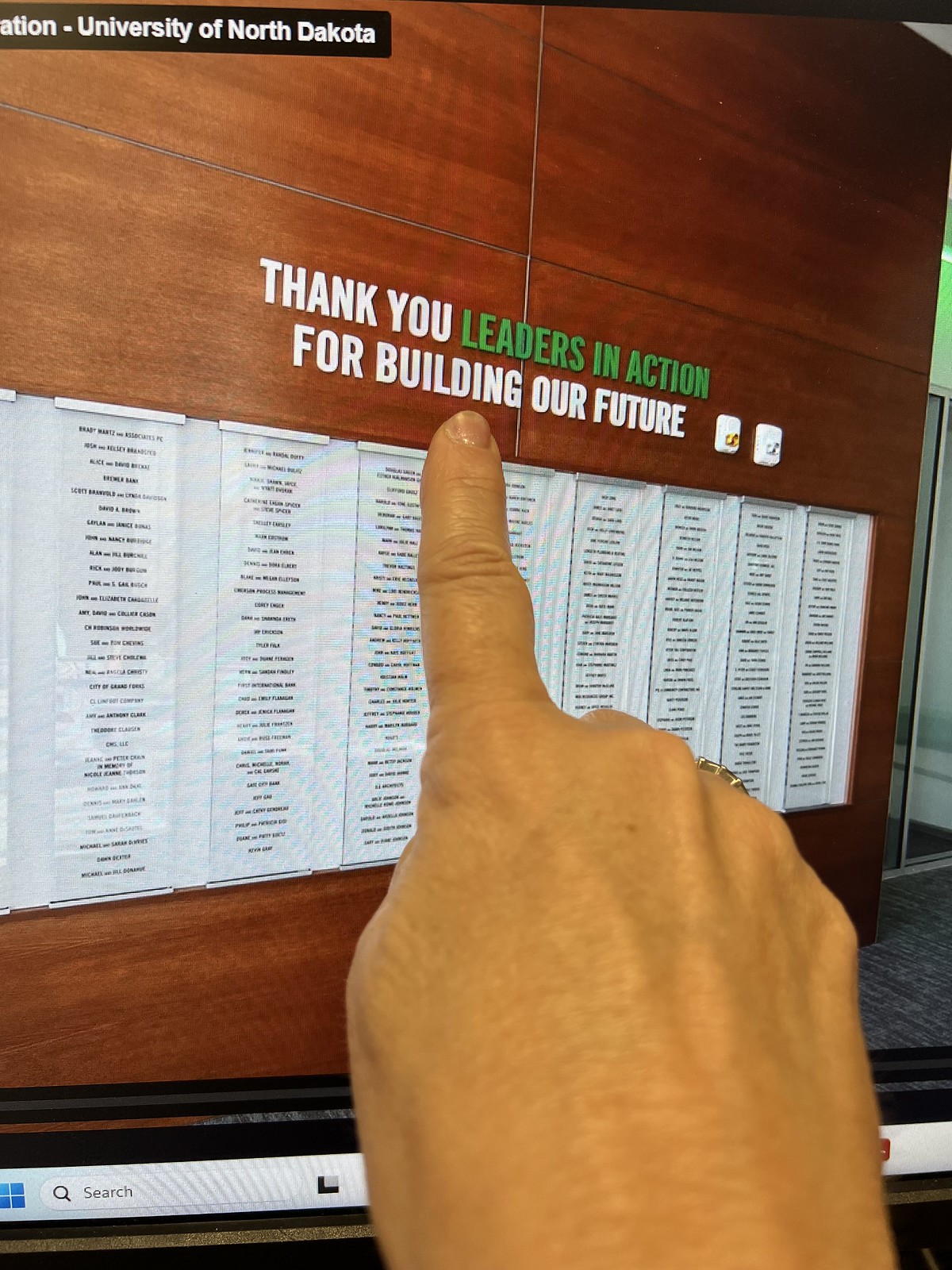The image is a photograph of a computer screen displaying a vertical, rectangular picture of a stained brown wood wall in an office environment, possibly at the University of North Dakota. On the wall, there is a large white plaque with dozens of names, organized in about seven or eight columns, appearing to honor individuals working in the building. Above the plaque, a prominent sign reads, "THANK YOU, LEADERS IN ACTION, FOR BUILDING OUR FUTURE," with "LEADERS IN ACTION" highlighted in green. A hand in the foreground, visible from behind and adorned with a ring, points to the word "BUILDING" on the sign. The image, visible on what might be a laptop, also shows a partial search bar at the bottom of the screen.